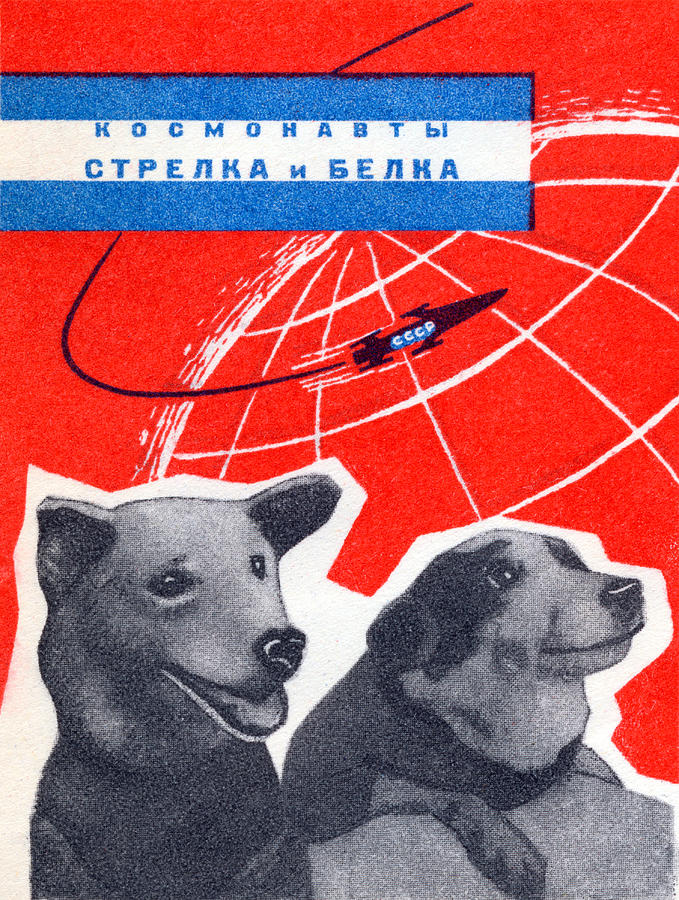This image appears to be a detailed cover, possibly of a book, magazine, or a graphic poster. Predominantly, it has a Soviet-era theme, featuring a vibrant red background with white longitude and latitude lines forming a globe at the center. Superimposed on this globe is an old Soviet rocket, black in color, with the lettering "CCCP" marked in white. Positioned above this, there's a blue and white striped flag with Russian writing, possibly spelling out "K-O-C-M-O-H-A-B-T" along with other characters. Below the globe and rocket, against a stark white background, are two black and white dogs, enclosed by a white border, seemingly gazing off to the side. One of the dogs is depicted perched on a gray rock, adding a layer of texture to the lower part of the image. Overall, this cover uses a combination of red, white, and blue hues to create a visually striking and narrative-rich illustration.